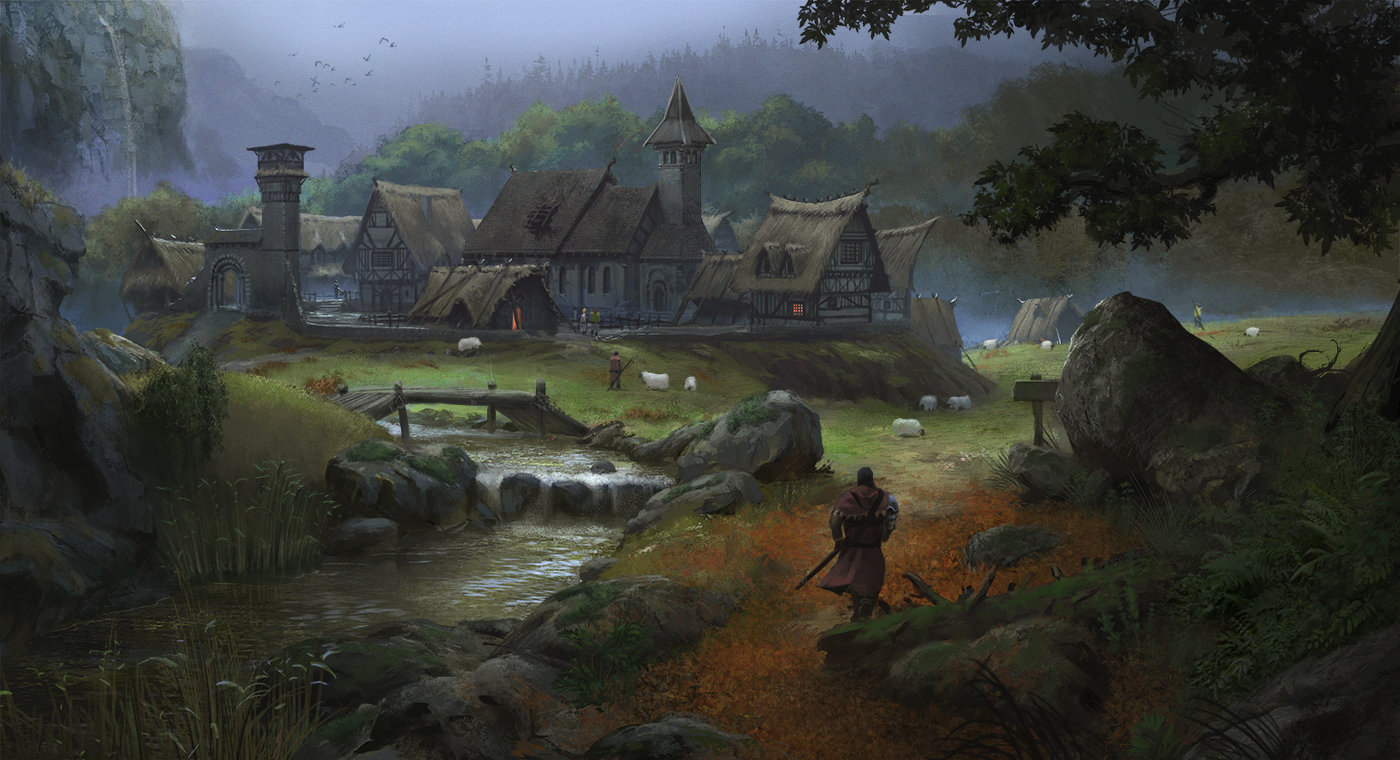This digital artwork, evocative of a European medieval scene, portrays a detailed and picturesque village landscape. In the foreground, a man clad in armor covered by a red robe walks along a riverbank, brandishing a sword in his left hand. The river, muddy gray in color, features rocky waterfalls, waves, and pockets of bubbles. A small wooden footbridge arches over the stream, surrounded by boulders and tall reeds. 

To the right, a thatched-roof cottage village perches on a small hill. This village, reminiscent of an old fortified base with most walls crumbled, still retains a main entrance and a lookout tower. The cottage structures are light gray or white with brown straw rooftops. There's also a group of sheep herders tending to white sheep in the fields around the village, with tents visible in the distance.

The serene landscape includes vivid greenery, blue skies, and soaring black birds. The background is marked by towering trees, mountains, and rocky cliffs with additional small waterfalls. The scene is shrouded in a misty, foggy atmosphere, enhancing the artistic and medieval ambiance.